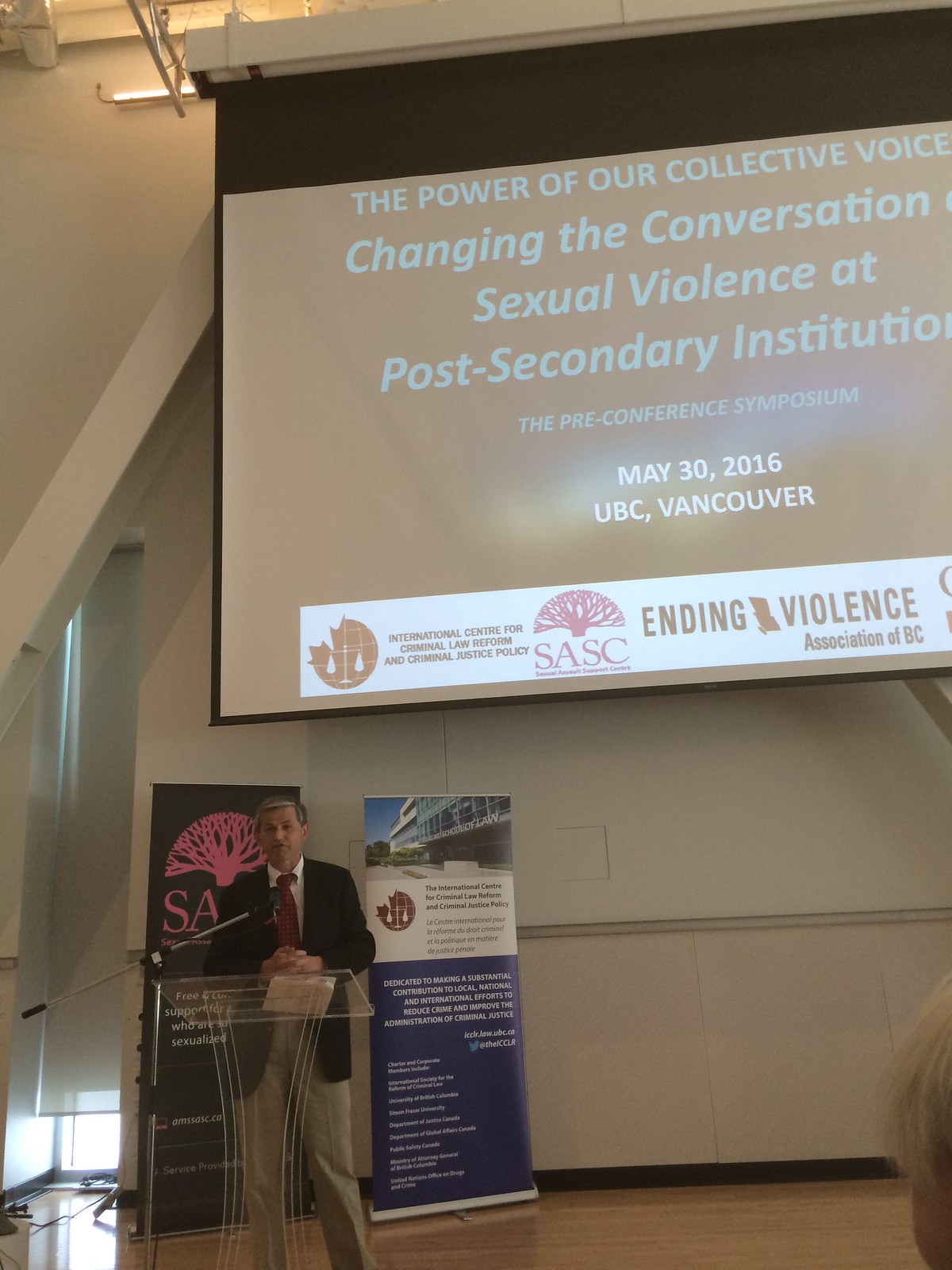The image captures a formally dressed man, wearing a black suit jacket, gray pants, a white shirt, and a red tie, standing at a white podium and speaking into a microphone. Positioned towards the bottom left of the image, the man is delivering a speech at a pre-conference symposium focused on "The Power of Our Collective Voice: Changing the Conversation on Sexual Violence at Post-Secondary Institutions." This event took place on May 30th, 2016, at UBC Vancouver. In the background, there are multiple posters in colors of white, blue, red, pink, and black, flanking both sides of the podium. The wooden floor occupies the bottom eighth of the image, while the remaining portion features the wall with a projector screen in the top right. Logos for various sponsors, including the International Center for Criminal Law Reform and Criminal Justice Policy, are visible on the screen, highlighting the event's collaborative nature. The overall setting suggests a well-organized academic or professional gathering aimed at addressing critical issues of sexual violence in higher education institutions.